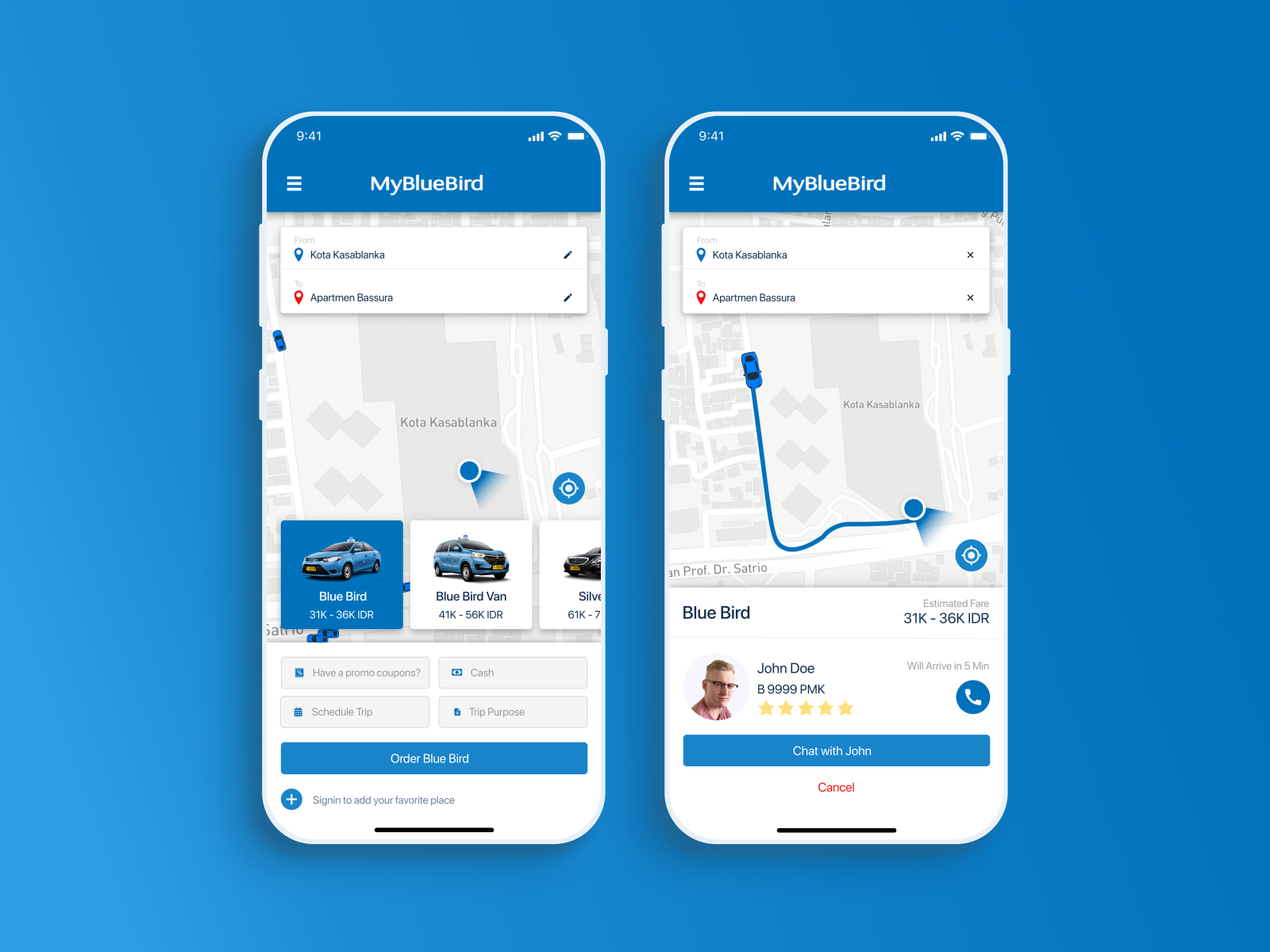The image depicts two smartphone screenshots side by side, each displaying the My Bluebird app against a solid blue background. Both screenshots indicate the app was accessed at 9:41 AM with a full battery charge of 100%. The top of the left screenshot prominently features the "My Bluebird" title.

In both screenshots, there's a small menu for searching or accessing a map, labeled with what appears to be the location "Coca-Coca-Burra, Aparambansara." The app content includes a list of services in a foreign language, likely related to transportation.

The left screenshot shows various vehicles available, suggesting either a car rental or purchasing service. Specific cars are listed with a price range of "31,000 to 36,000 IDR" (Indonesian Rupiah). 

At the bottom of each screenshot are two blue rectangular buttons: one labeled "Order Bluebird" and the other "Chat with John," indicating options for engaging with the service or customer support.

Overall, the app appears to provide transportation or vehicle rental services in a non-English language, specifically referencing Indonesian currency (IDR).